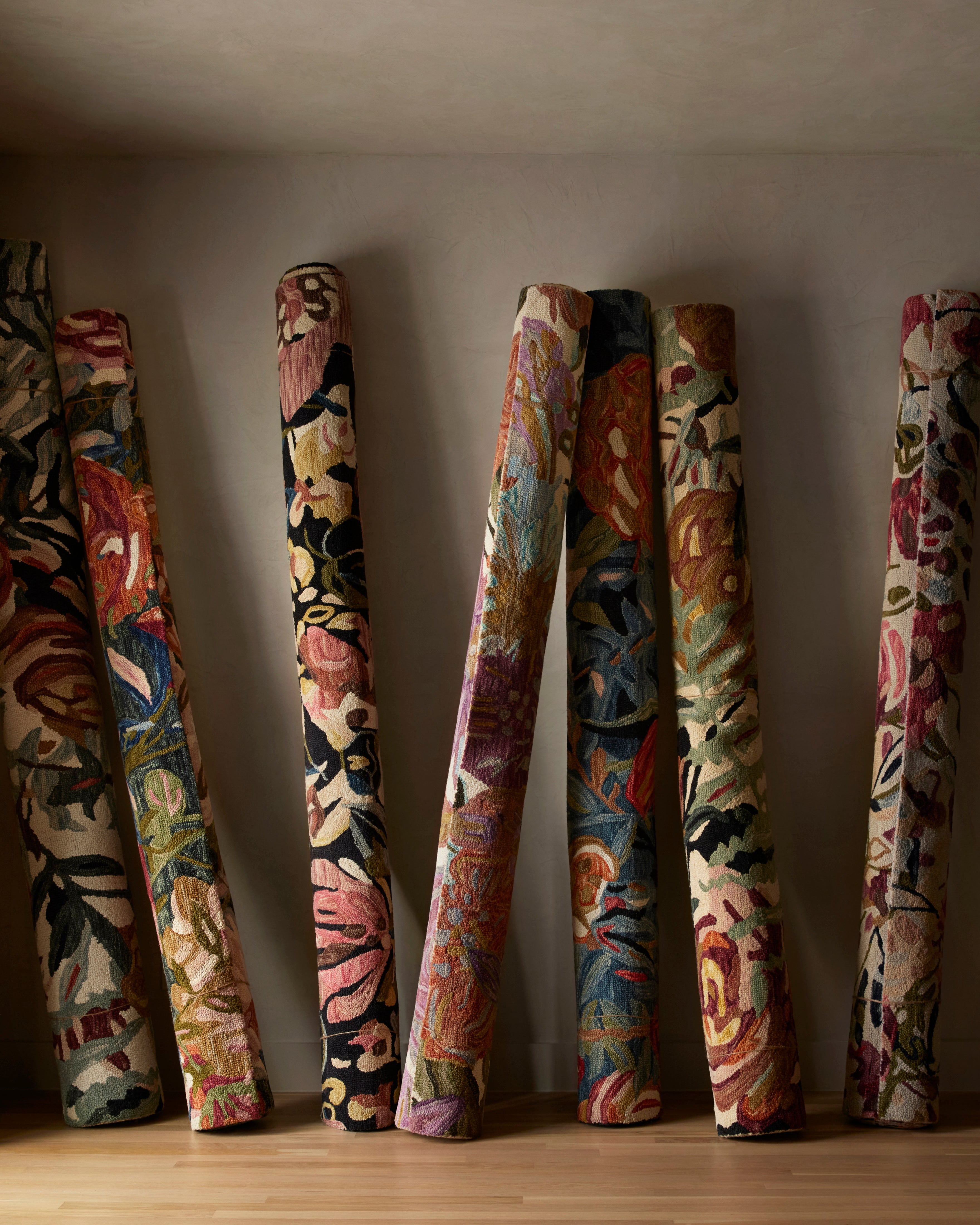The photograph showcases seven large, rolled-up rugs or tapestries, all vibrant and colorful with bold, floral, and paisley designs. These rolls are leaning against a plain, beige wall and positioned on a wooden floor made up of horizontally-oriented light-colored planks. From left to right, the first rug, which is slightly off-camera, features maroon, green, and beige hues. The second rug sports green, blue, red, and beige tones, followed by a black, red, gold, and white rug. The overall palette includes striking pinks, oranges, blues, and blacks, with intricate patterns of flowers and leaves visible only around the curved edges of the rolled rugs. Additionally, one roll in the center rests against another, suggesting an additional dimension of arrangement. There is a light source illuminating the scene from the left, adding a subtle shine to the vibrant, organic patterns of the rugs.